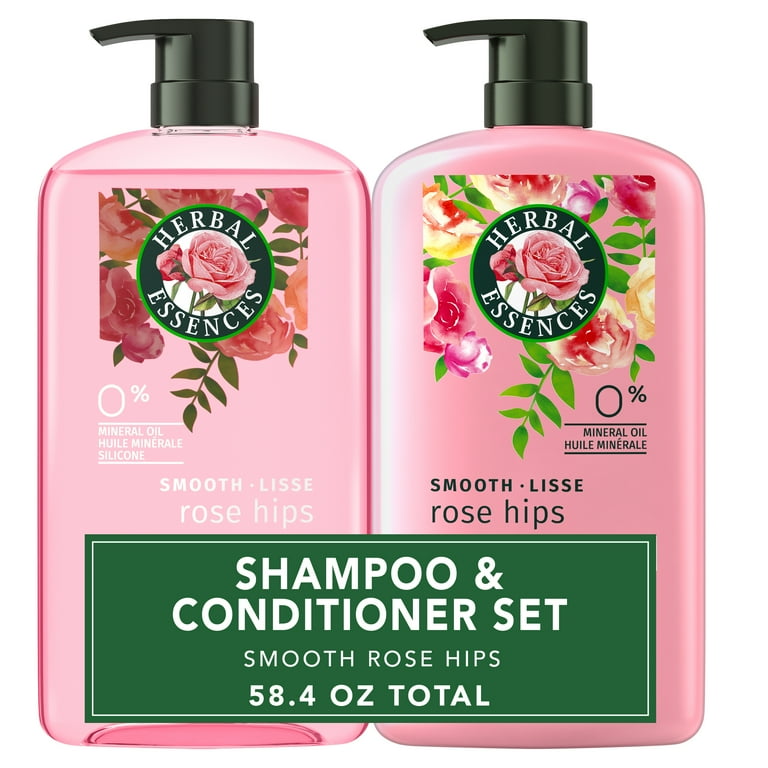The image features a set of shampoo and conditioner from Herbal Essences, showcasing two bright pink bottles with black pump tops. Each bottle is adorned with a floral design that prominently features pink roses surrounding the Herbal Essences logo. The label on the bottles indicates that the variety is "Smooth Rose Hips" and confirms they contain 0% mineral oil. In front of the bottles, a green banner clearly states, "Shampoo and Conditioner Set, Smooth Rose Hips, 58.4 ounces total" in white text, further accentuating the cohesive packaging design. Additional text on the packaging appears to be in both English and French, detailing the product's ingredients and benefits.